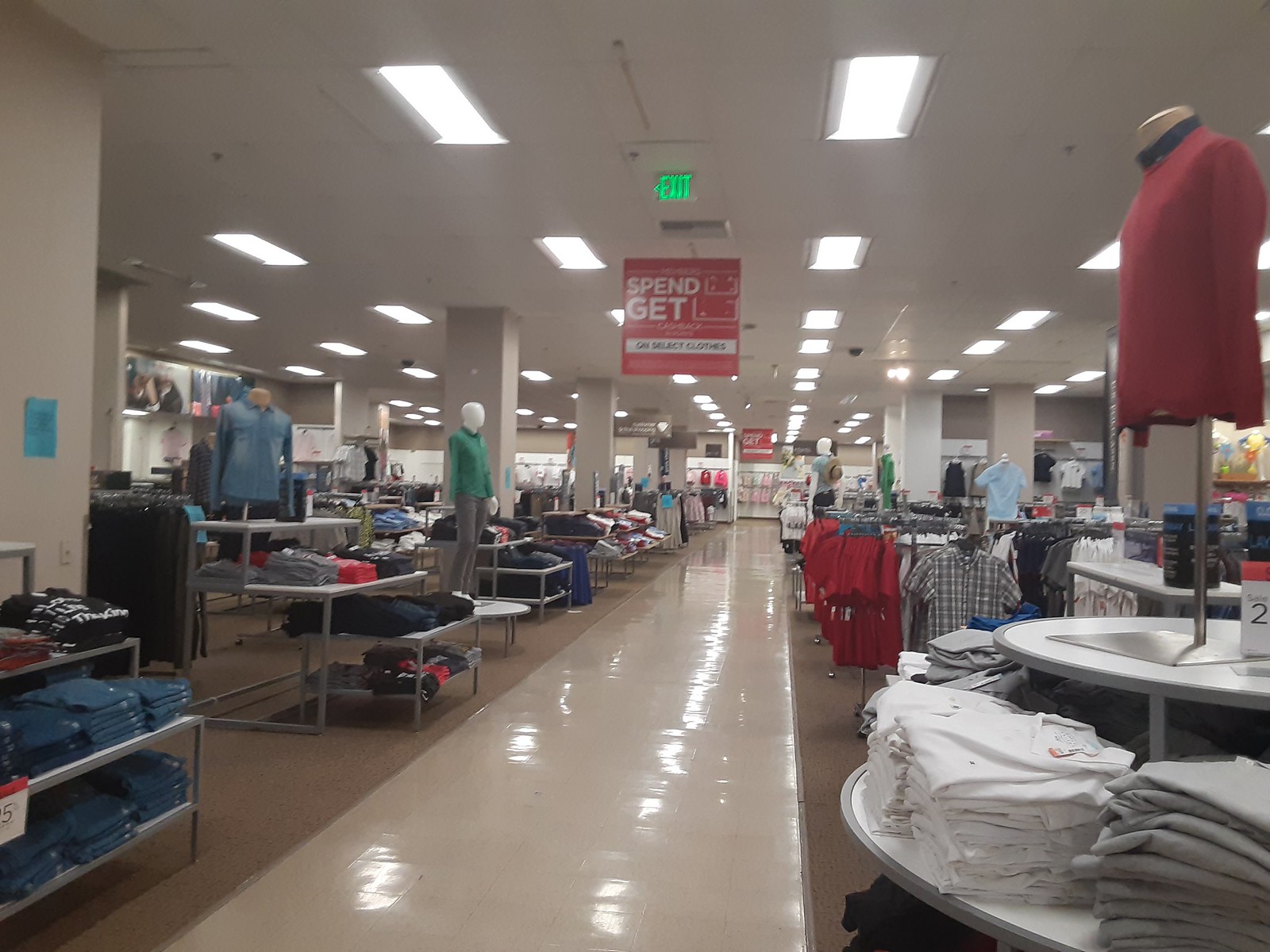The image depicts the well-lit interior of a major department store, resembling JCPenney or Macy's. The scene is centered on a highly polished, shiny, off-beige linoleum walkway that runs towards the back of the store. Flanking this walkway are carpeted sections, characterized by light tan industrial carpeting. On the right side, there are circular stands with neatly folded shirts, including a prominent red long-sleeved shirt displayed on a headless mannequin on a metal stand. Surrounding this display are additional piles of folded shirts and freestanding metal racks showcasing a variety of button-up, plaid, and other men's shirts, creating a diverse clothing area that extends further into the store.

On the left side, the setup mirrors the right, featuring tiered shelves and racks filled with more clothing items, accompanied by mannequins – some full-bodied and others just partial forms. A notable sign hangs from the white fluorescent-lit ceiling, displaying the partially obscured message on a red background with white text: "Spend... get... on select clothes." Additionally, a green exit sign with an arrow pointing the way out is visible in front of this promotional sign.

The store's layout emphasizes the organized presentation of men's clothing, highlighted by folded jeans, structured displays, and ample product variety.